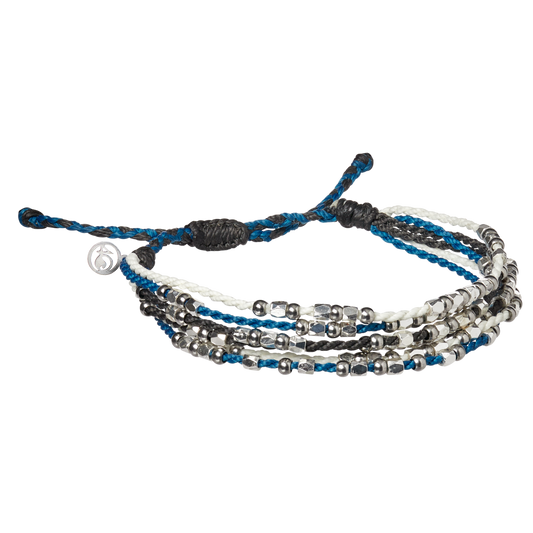This image depicts a handmade bracelet set against a white, borderless background. The bracelet consists of five tiers comprising strings of white, blue, and black hues. Intertwining and braided, these strings are adorned with alternating sections of silver and clear beads, creating a repeating pattern. The strings tie together at the back with a black knot, where a small silver charm featuring a swirly coin design is attached. The silver beads vary in shape, with both round and square beads present. The photo is taken from a slight downward angle, providing a comprehensive view of the intricate detailing and craftsmanship of the bracelet.